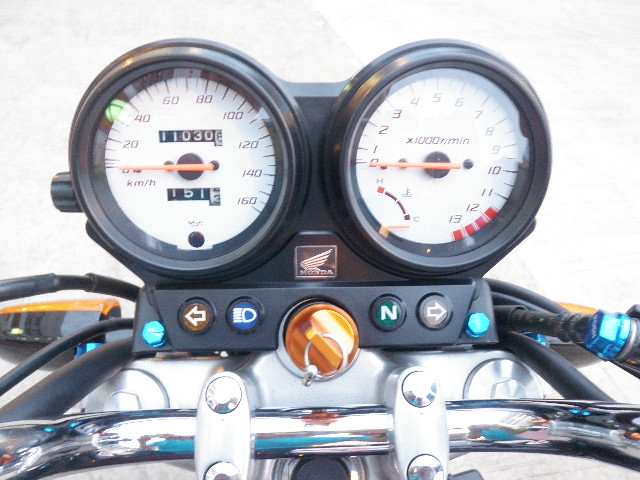A detailed image shows the odometer and tachometer of a motorcycle, specifically of a Honda brand. The left circular dial, encased in a black rim, features a white face with black numbers incrementing from 0, 20, 40, 60, 80, 100, 120, 140, up to 160. This dial also has vibrant orange hands indicating specific values. Located at the top center within this left circle, the odometer display reads "110308" (though the last digit is partially obscured). Directly below the needle, a trip meter displays "1513".

The right circular dial, also with a white face and black numbers, measures revolutions per minute (RPM), marked from 0 up to 13 (x1000 RPM). It too has an orange hand, and above this hand, the label "X 1000 R per minute" is visible. A small red square marked with an "H" is positioned in the bottom left corner of this dial, connected by curved lines to a black square labeled with a "C".

Between the two dials is the iconic Honda emblem, featuring a wing-like symbol. Directly below the emblem appears a key ignition surrounded by an orange-colored ring with an attached keyring. Further down, several indicator lights are visible, likely denoting turn signals and various drive settings. The lower part of the image reveals a glimpse of the motorcycle's silver metallic body.